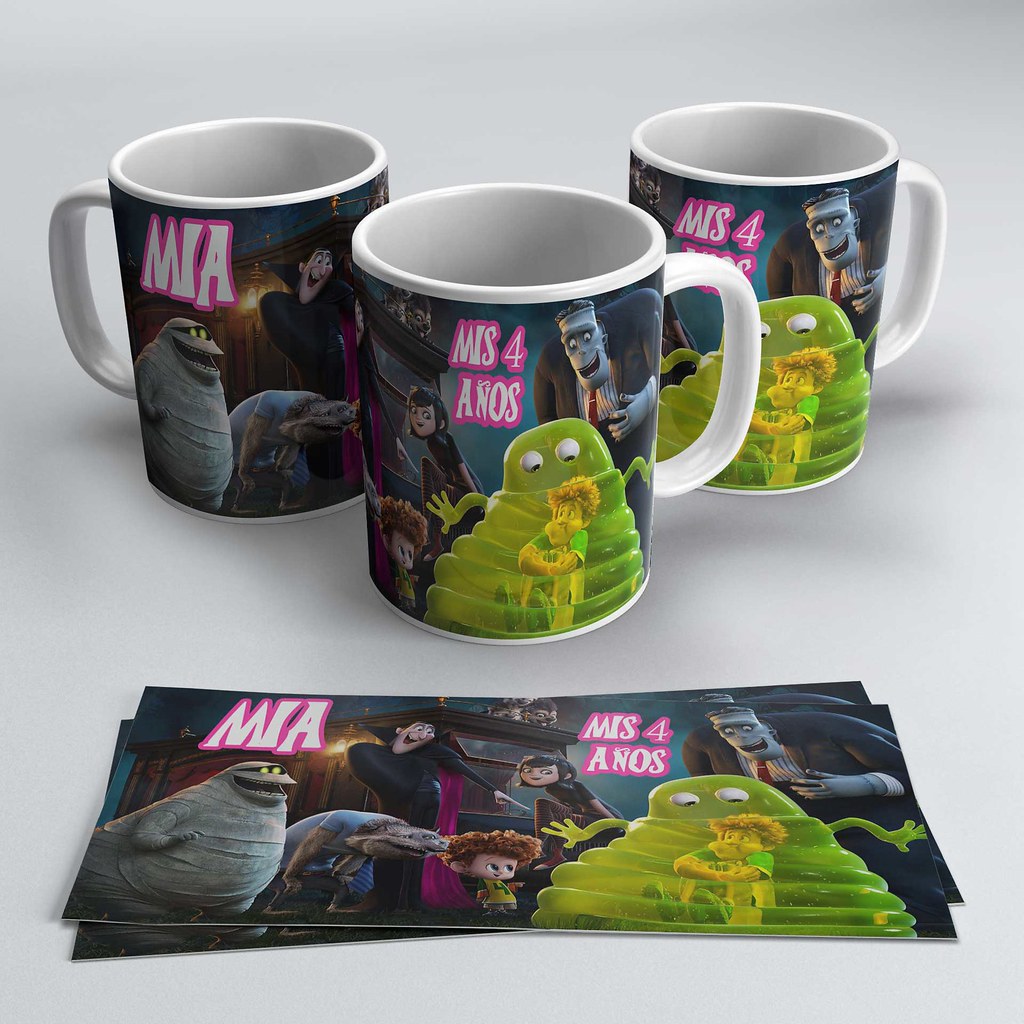This advertising photograph displays a set of vinyl wraps designed for coffee cups, themed around the movie "Hotel Transylvania." Against a plain white background, three white ceramic mugs stand side by side, each wrapped with a vinyl skin showcasing the film's iconic characters. The wraps feature vibrant illustrations of a Frankenstein-style monster, a vampire, a green jello-like blob monster, a mummy, and a girl with black hair. Additional details include the text "Mia - Mis 4 Años," indicating a fourth birthday celebration in Spanish.

In front of the mugs lies a neat stack of the same vinyl wraps, ready to be applied. This photo embodies the festive spirit, hinting at a party gift set, perhaps aimed at a young "Hotel Transylvania" fan named Mia. The bright and fun designs suggest an engaging, themed birthday experience for children, blending practicality with the joy of personalized party favors.